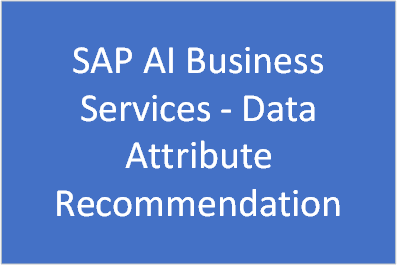In this rectangular image set against a light blue background, a solid blue rectangle resembling a business card is prominently displayed. The rectangle features the following text in large, bold white font: At the top, the phrase "SAP AI Business" is written. Directly beneath it, the word "Services" is centered. Below "Services," the word "Data" is placed. Centered under "Data" is the word "Attribute," and finally, at the bottom of the rectangle, the word "Recommendation" is displayed. The text is simple and clearly laid out, providing a clean and straightforward visual of the key terms related to SAP AI's business elements.